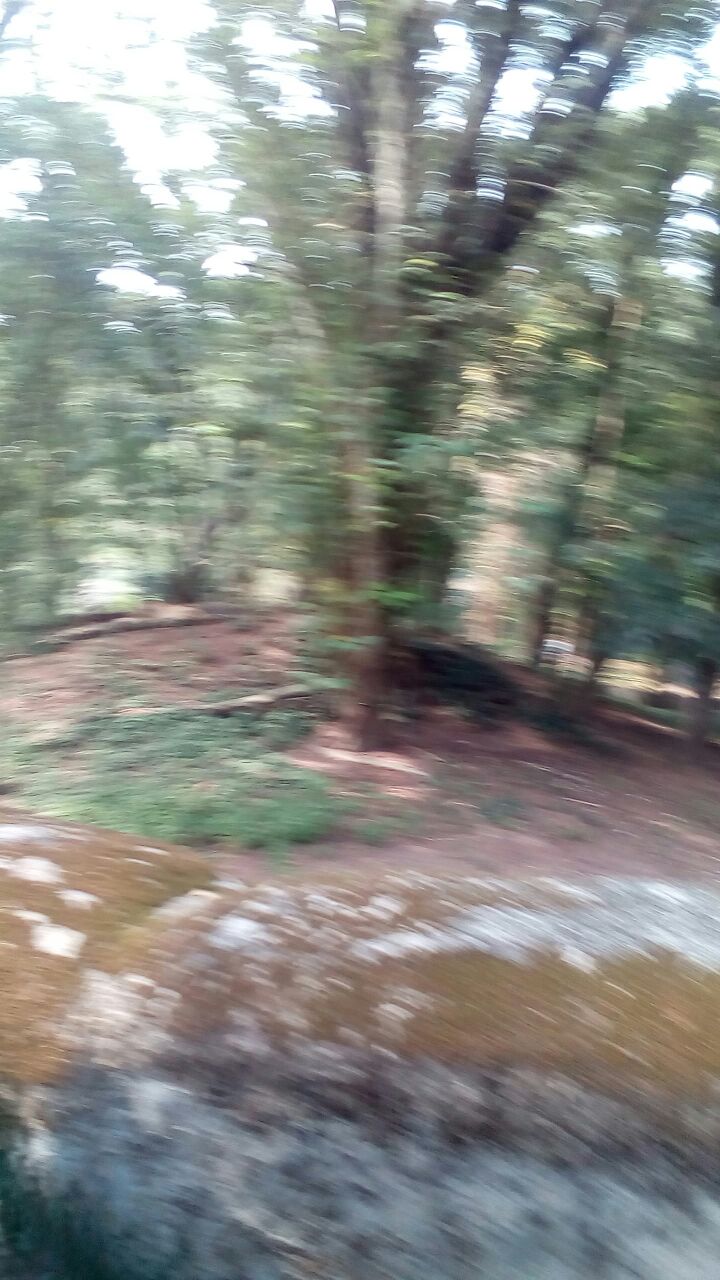A blurry photograph taken in a forest captures an indistinct scene that appears to feature an animal. The image shows a dense backdrop of trees bathed in sunlight, with patches of grass and dirt on the forest floor. The likely presence of a small, four-legged animal with a long tail, possibly a fox, can be discerned near the lower left side of a central tree trunk. The animal seems reddish in color, though the blurriness makes it hard to be certain. At the bottom of the image, there is an unclear, dark grayish area with what could be a liquid surface above it, adding to the enigmatic nature of the scene. Despite the difficulty in making out specific details, the photograph exudes a natural, sunlit woodland atmosphere with a hint of mystery about the exact subject captured.